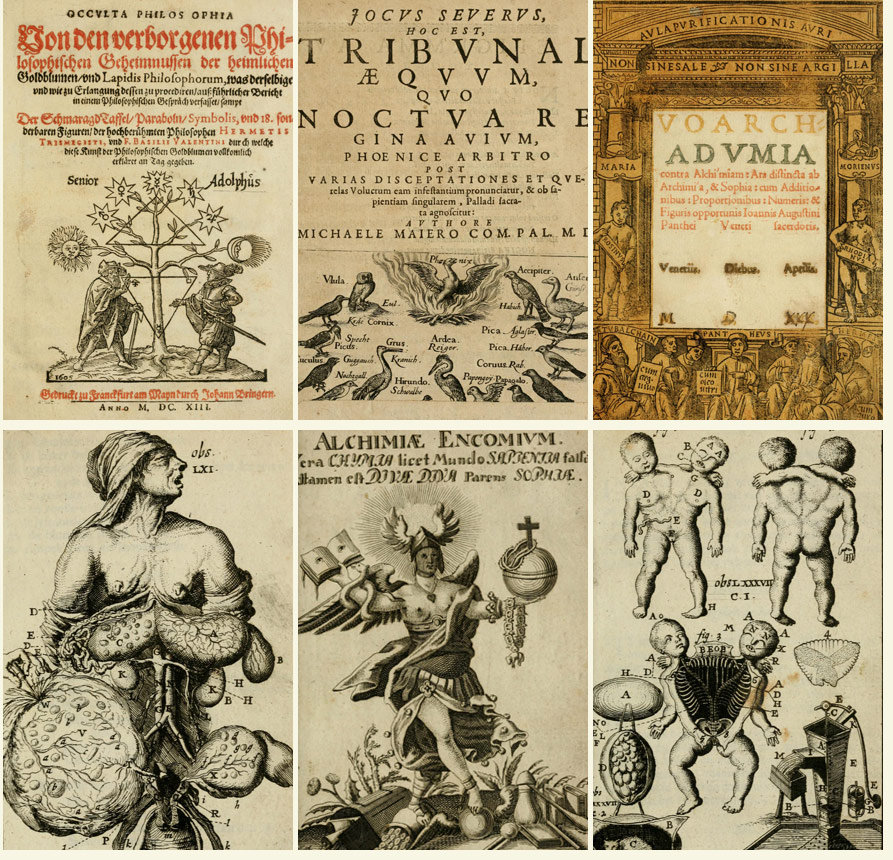The image is a composite of six detailed photographs from what appears to be an ancient manuscript, likely written in Latin. The top left segment features an illustration with red and black text, depicting two men flanking a tree adorned with male and female symbols on its stars. Adjacent to this, in the top middle, is an intricate drawing of various bird species arranged in a circle. The top right section, rendered in a golden hue, contains the cover of the book, showcasing the quality of its aged paper. On the bottom left, there is a detailed depiction of a figure, possibly an androgynous human, with an exposed chest and bulbous formations covering the lower body. The bottom middle illustration portrays a man holding a globe and cross in one hand and a book in the other, symbolizing knowledge and authority. The bottom right segment provides a striking image of conjoined twins, shown frontally, from the back, and with their internal anatomy visible. The entire composition suggests themes of alchemy or the occult, underscored by the intricate, hand-drawn illustrations and the ancient, somewhat eerie nature of the text and images.